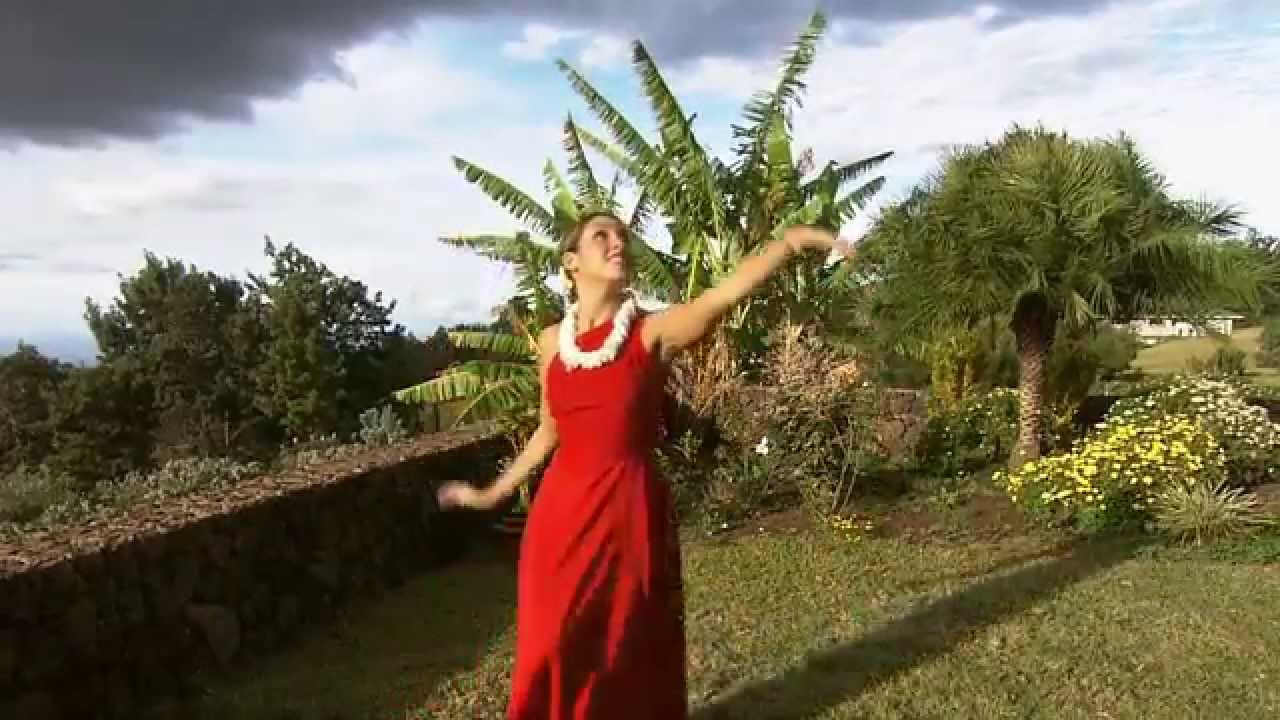In this vibrant outdoor photograph, a woman is gracefully posed as if dancing in the midst of a lush garden. She is adorned in a full-length red dress that flows elegantly around her. A white garland decorates her neck, adding a touch of purity to her striking appearance. With her arms spread wide and her head tilted upwards to the upper right, she exudes a sense of freedom and joy. The ground beneath her feet is a carpet of green grass, and surrounding her, in the front and left, is a dark brown border fence that frames the scene. The foreground of the garden is lush with various plants and trees, adding depth and richness to the setting. Above, the sky is a canvas of blue, interspersed with a mix of white and dark grey clouds, suggesting a dynamic, ever-changing weather.